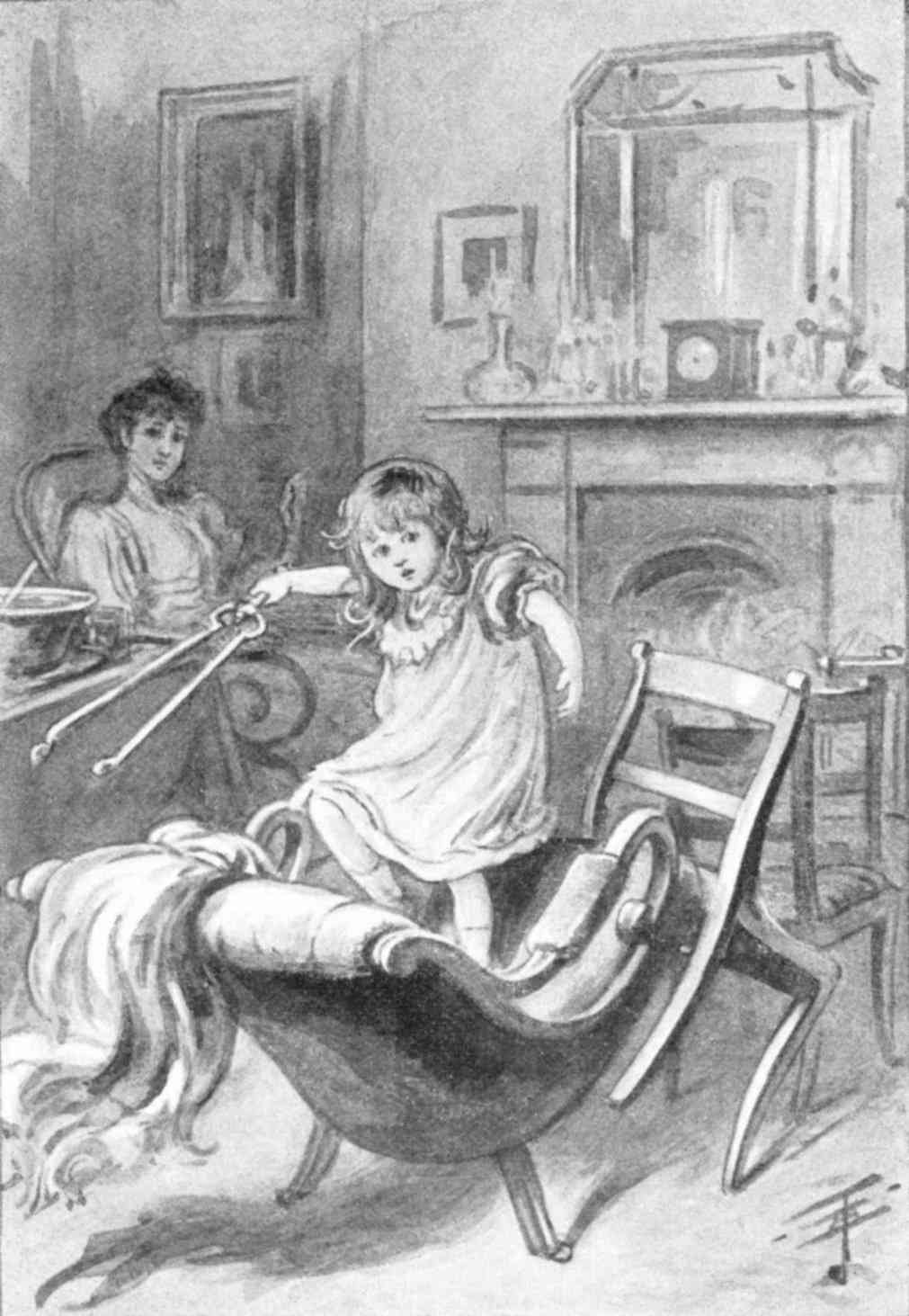This detailed black and white pencil drawing depicts an interior scene from the 1800s to early 1900s. At the center, a woman dressed in an old-fashioned gown with her hair styled up and bangs is seated in a rocking chair. Beside her, a young girl, possibly her daughter, is standing precariously on a chair held up by another tipped chair. The girl, attired in a nightdress and with long hair, holds a pair of tongs and gazes toward the viewer with an uncertain expression. The scene is set against the backdrop of a cozy home with a fireplace, a mantel adorned with an old-school clock, a vase, and a mirror, along with three framed pictures or paintings. A blanket drapes over the chair supporting the girl, and a bowl sits next to the seated woman, adding to the domestic atmosphere.